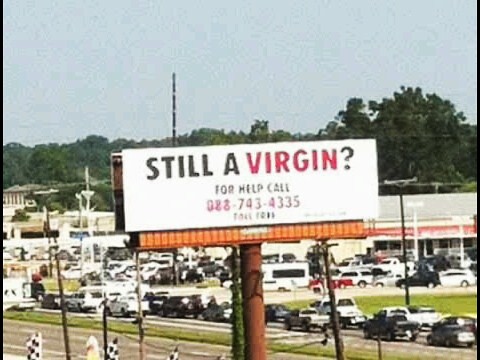This photo, seemingly taken decades ago due to its low resolution, captures a striking street scene centered around a billboard. The billboard, with its white background, prominently displays the message "Still a Virgin" in a dramatic mix of black and red text, along with a phone number for assistance. The words "still a" are in black, while "virgin" is highlighted in red. 

In the foreground, the bottom left corner of the image shows a snippet of a street, bordered by a patch of grass. Adjacent to this, a street with two to three lanes is visible, filled with a lineup of primarily black, white, and gray cars. Further in the background, beyond another strip of grass, lies another street also populated with vehicles. 

Dominating the mid-ground is a parking lot leading up to a shopping center. The shopping center features large glass doors and windows, and one can discern a red sign presumably displaying the store name, although the details are not entirely clear. Topping the scene off, a roof structure is evident, framing the background of leafy trees and an expansive sky.